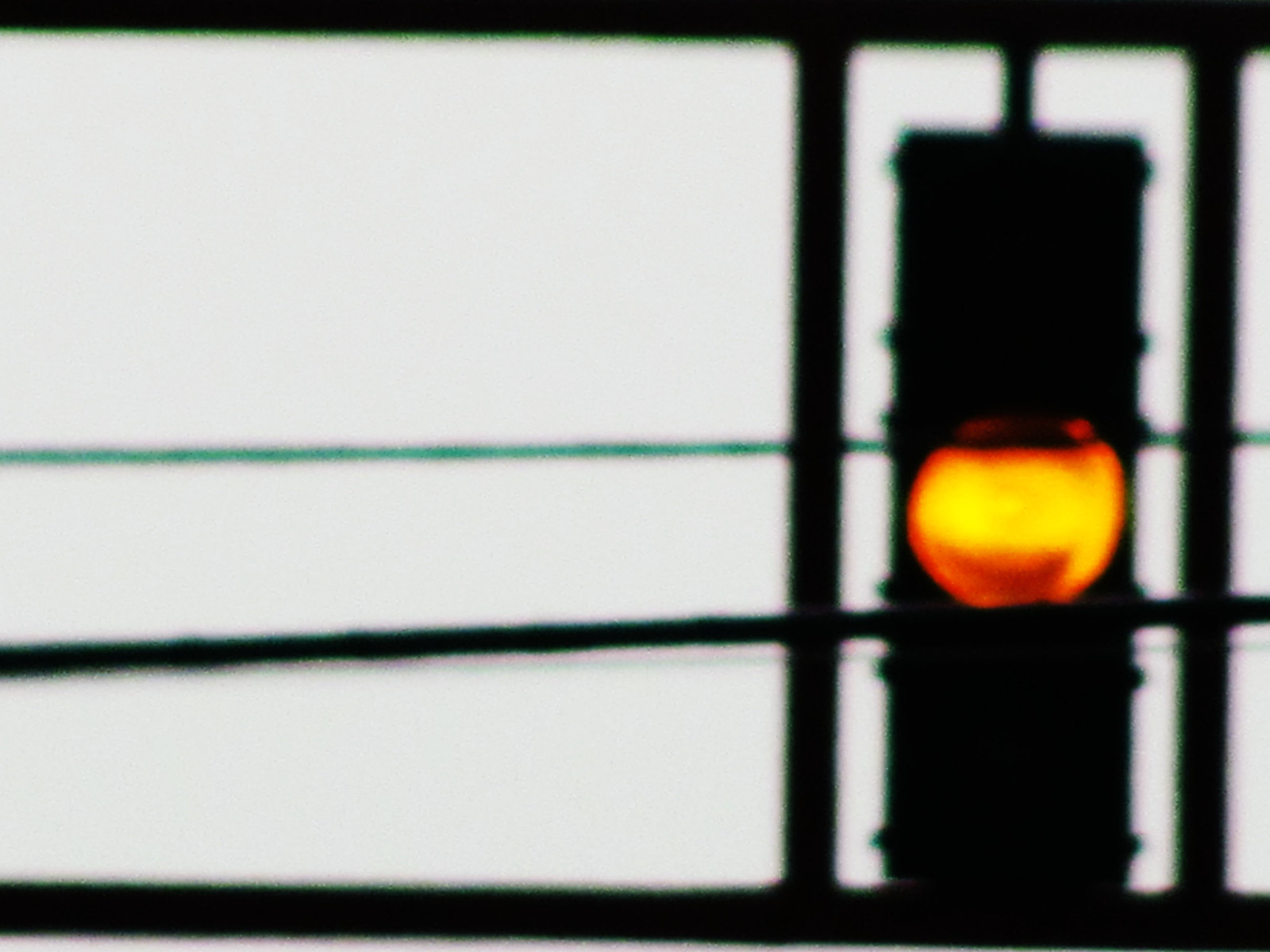A slightly blurry photograph captures a streetlight with three distinct sections, with the central yellow light illuminated. The streetlight is partially obscured by an indistinct object in the foreground. It appears to be photographed through a window or similar barrier, adding an additional layer of distortion to the image. The top section of the streetlight is visible, extending out of the frame and suggesting connection to an overhead support structure. The background has a bluish tint, further contributing to the photograph's hazy appearance.